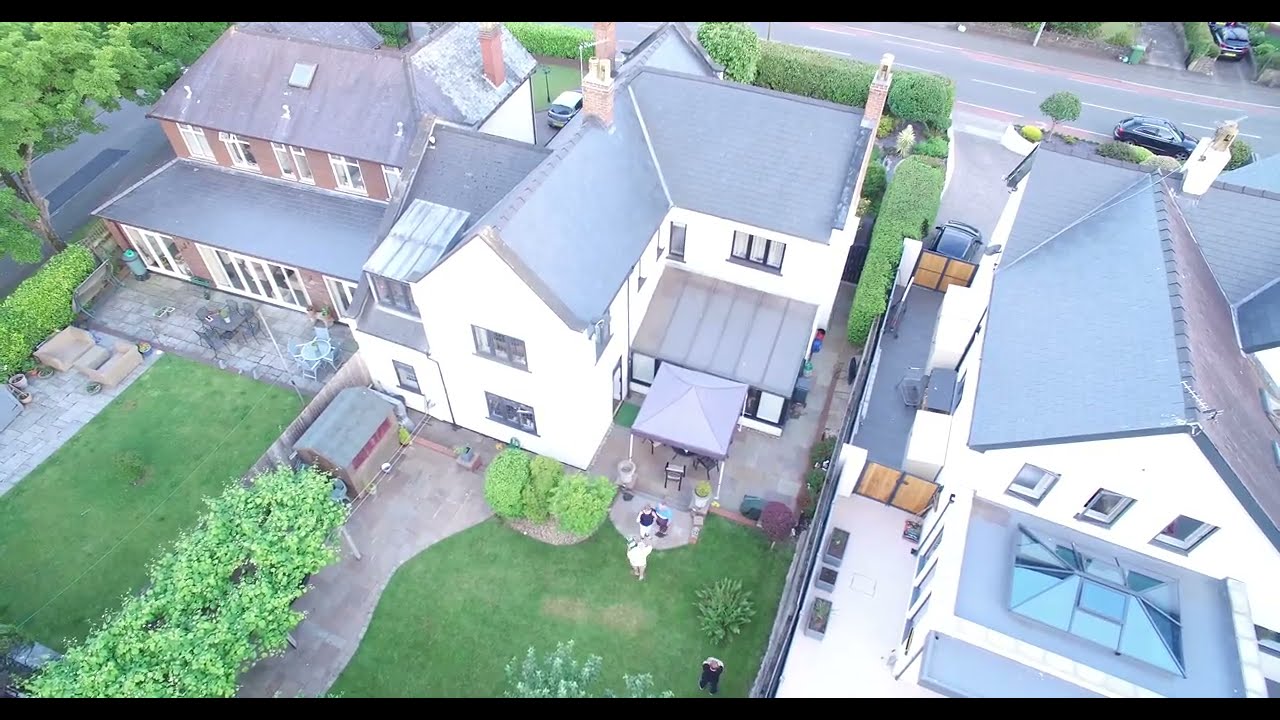This is an aerial view, likely taken from a drone, showcasing three houses in a neighborhood. The image captures the backyards prominently, while the street with parked cars runs along the top edge in the background. The houses are primarily white with black roofs, and the yards are meticulously maintained with cut grass and various landscaping details.

From left to right:
- The first house is a two-story, older-style building with a brown exterior. The backyard features a walkout patio furnished with patio furniture and stone paths amidst a small grassy area. A single car is visible in the driveway.
- The middle house, also two stories and white, has a more built-out patio with a covered top. The backyard is lively, with a family (potentially two kids, a wife, and a husband). There is a shed, well-kept grass, a concrete walkway, and a porch area covered by a canopy. A large grill is nestled in the corner of the flagstone patio.
- The third house, partially visible, exudes a modern look with a white exterior and black roof. Its backyard is predominantly paved, with minimal greenery. There's a car with its doors open in the driveway.

The image’s color palette includes whites, blacks, browns, brick reds, grays, greens, and blues, adding vibrancy to the detailed scene.